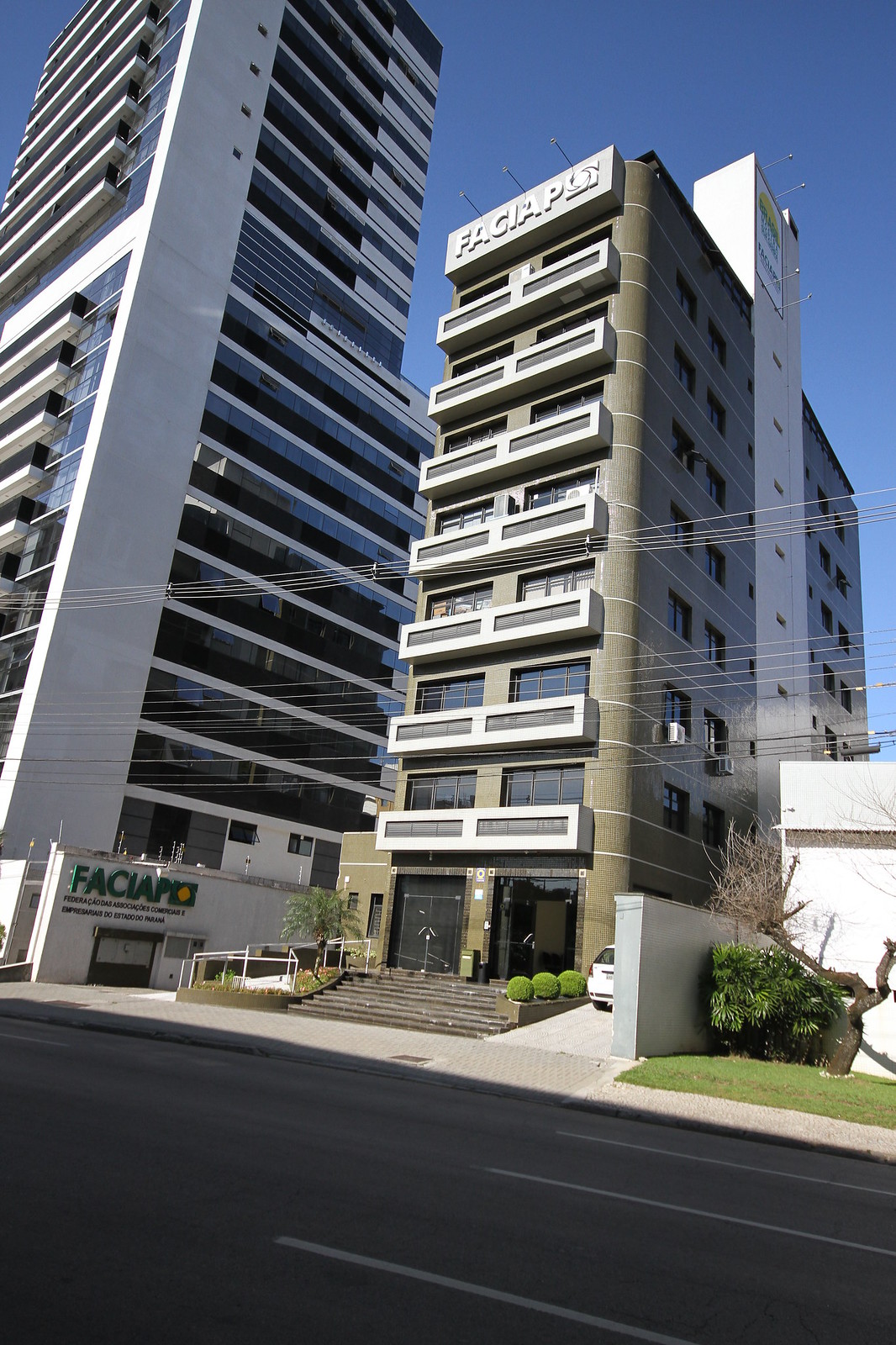The image features a daytime photograph of two distinct buildings, viewed from ground level. The main focus is on a building named Fakhiapos, which stands 8 stories tall. This structure includes several sets of windows and what appears to be a patio area. In the foreground, there is a road with black asphalt and white lines, and a newer white or yellow vehicle, possibly parked in a driveway area next to the building. A small stairwell with approximately 10 steps leads to the entrance of Fakhiapos. To the left of Fakhiapos is a significantly taller white building of a completely different design, also named Fakhiapos. The scene includes a cement wall with bushes separating Fakhiapos from the adjacent business, suggesting this is not a location in America. Overhead, electrical wires run from left to right, and there is clear blue sky, indicating it is daytime. The photograph includes several identifying features like the name of the building and surrounding elements such as the road, sidewalk, and partial views of a neighboring small building and shrub.